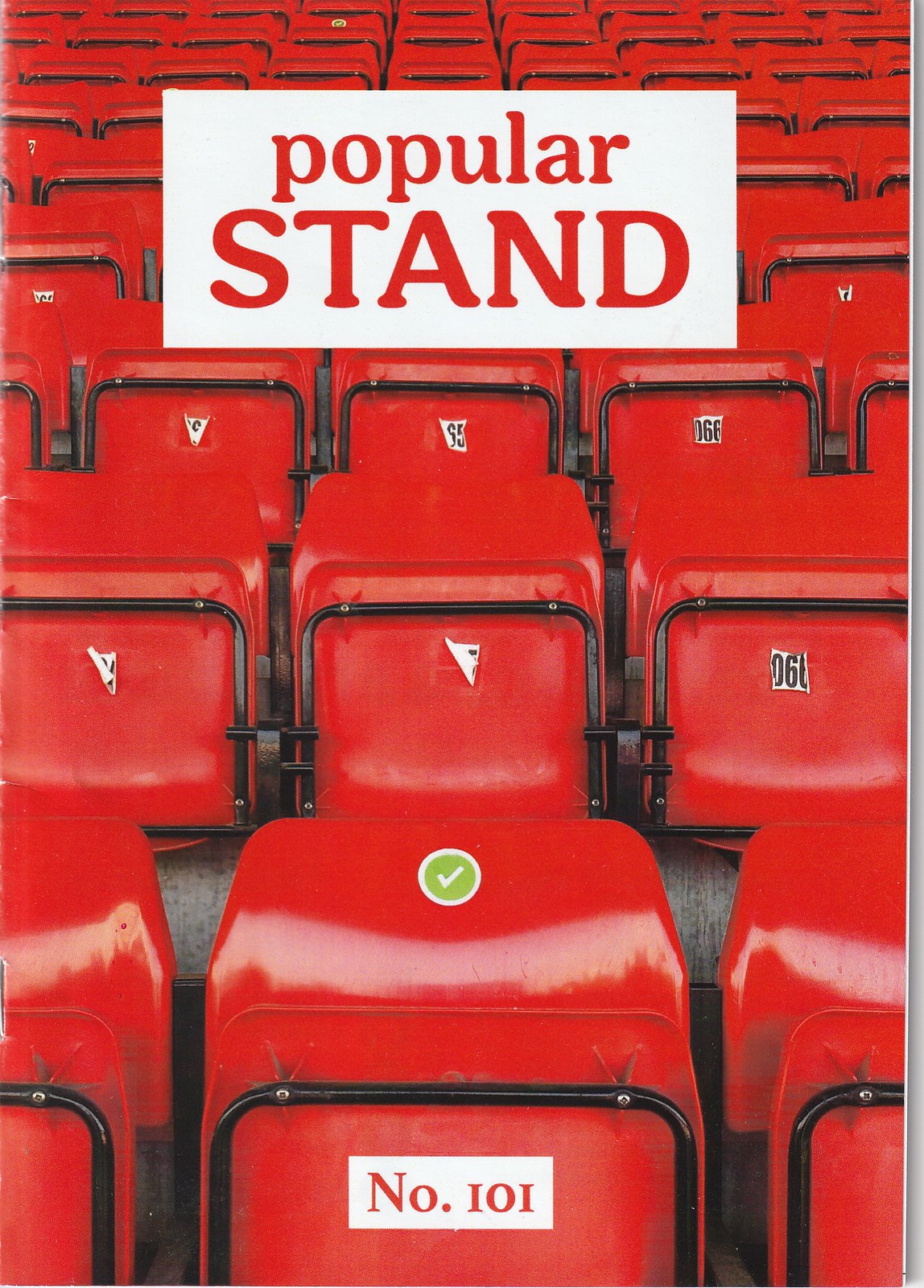This image showcases a series of red folding stadium seats, arranged in tidy, uniform rows. The chairs are all folded up flat, revealing a pattern of black-framed seats fixed onto a concrete base, which gradually become more numerous and smaller as they extend from the bottom to the top of the frame. There are also visible numbers on the seats, often displaying “65” or “66”, with one exception at the bottom center where a seat is marked with the number “101” in a white triangle. Just above this seat, there is another seat marked with a green circle containing a white check mark. At the top of the image, a white text box with red font reads "popular stand," with "stand" capitalized, indicating a probable magazine cover format. The image is devoid of any other objects, focusing entirely on these neatly arranged stadium seats.